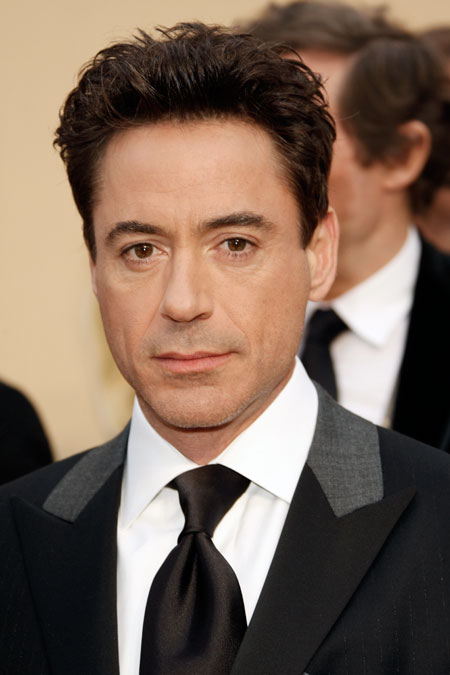The photograph features a man who closely resembles actor Robert Downey Jr., with dark brown, gelled hair that appears layered and slightly spiked. He has dark brown eyes and dark eyebrows, and his complexion is pale. He is dressed in a formal black suit jacket with contrasting light gray on the lapels, a white collared button-up shirt, and a pure black tie, suggesting he is attending a fancy event. The man is looking directly at the camera in a close-up shot. In the background, you can see another person, also dressed in formal attire with a black top, white shirt, and black tie, though only their brown hair, ear, and shoulder are partially visible. Overall, the detailed and well-composed elements of the scene create an atmosphere of elegance and sophistication.